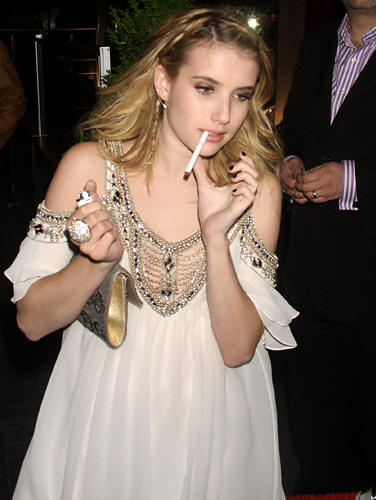The image captures actress Emma Roberts in a detailed and elegant ensemble. She is wearing a white dress adorned with intricate embroidery, gems, and jewels on the top, which features shoulder cutouts and straps. Her dress transitions into fluffy sleeves and a V-neckline embellished with rhinestones. Emma's blonde hair appears slightly disheveled, giving her a effortlessly chic look. In her right hand, she holds a lighter and a clutch decorated with gold, silver, and butterfly designs while showcasing a large, circular silver ring on her middle finger. A white cigarette hangs from her mouth, and her left hand is raised towards her chin. Her nails are painted black. Behind Emma, a man in a black suit with a white striped shirt in blue or purple stands to her right, though his face is out of the frame.